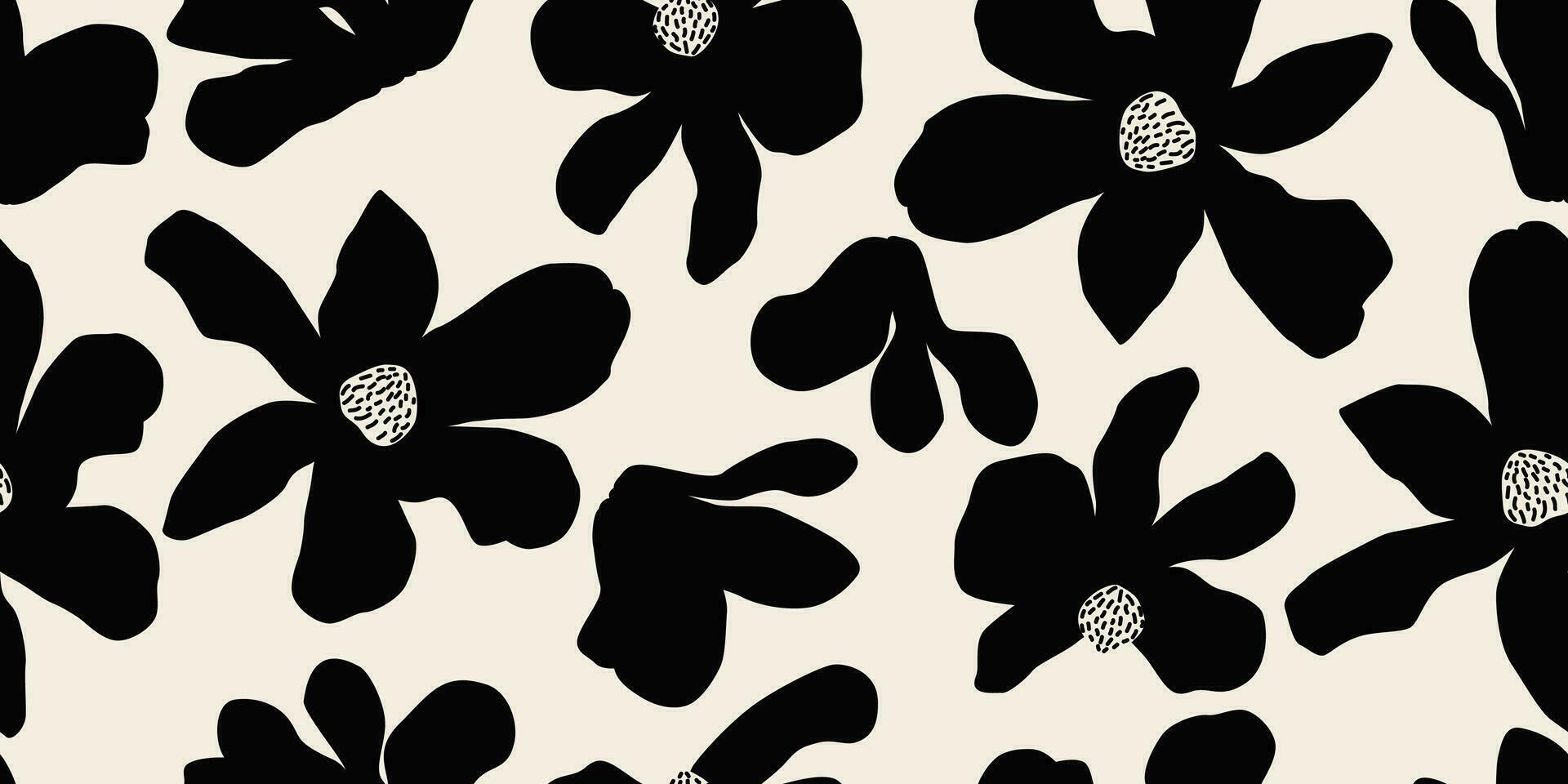This is a high-contrast, black-and-white rectangular digital illustration with an off-white background, resembling a vector image likely created in Illustrator. The pattern features black silhouettes of flowers, with each flower's bulb represented as a white, somewhat lumpy circle adorned with small black dots and dashes, adding texture. These flowers vary in size and orientation, with petals displayed at different angles. Most flowers have six petals, though some have three or four. The overall layout suggests a repeatable pattern, with the left and right edges aligning well for potential textile design, though it's not perfectly tileable. At the top, there are two large flowers with white centers, partially cut off by the image's edge. In the middle left, the largest visible flower has six petals and a white center. To its right, there's a smaller five-petaled flower with a white center, and further right, another flower with a visible center is partially cropped by the image's boundary. The flowers' leaves are depicted facing various directions, emphasizing their natural, irregular arrangement.